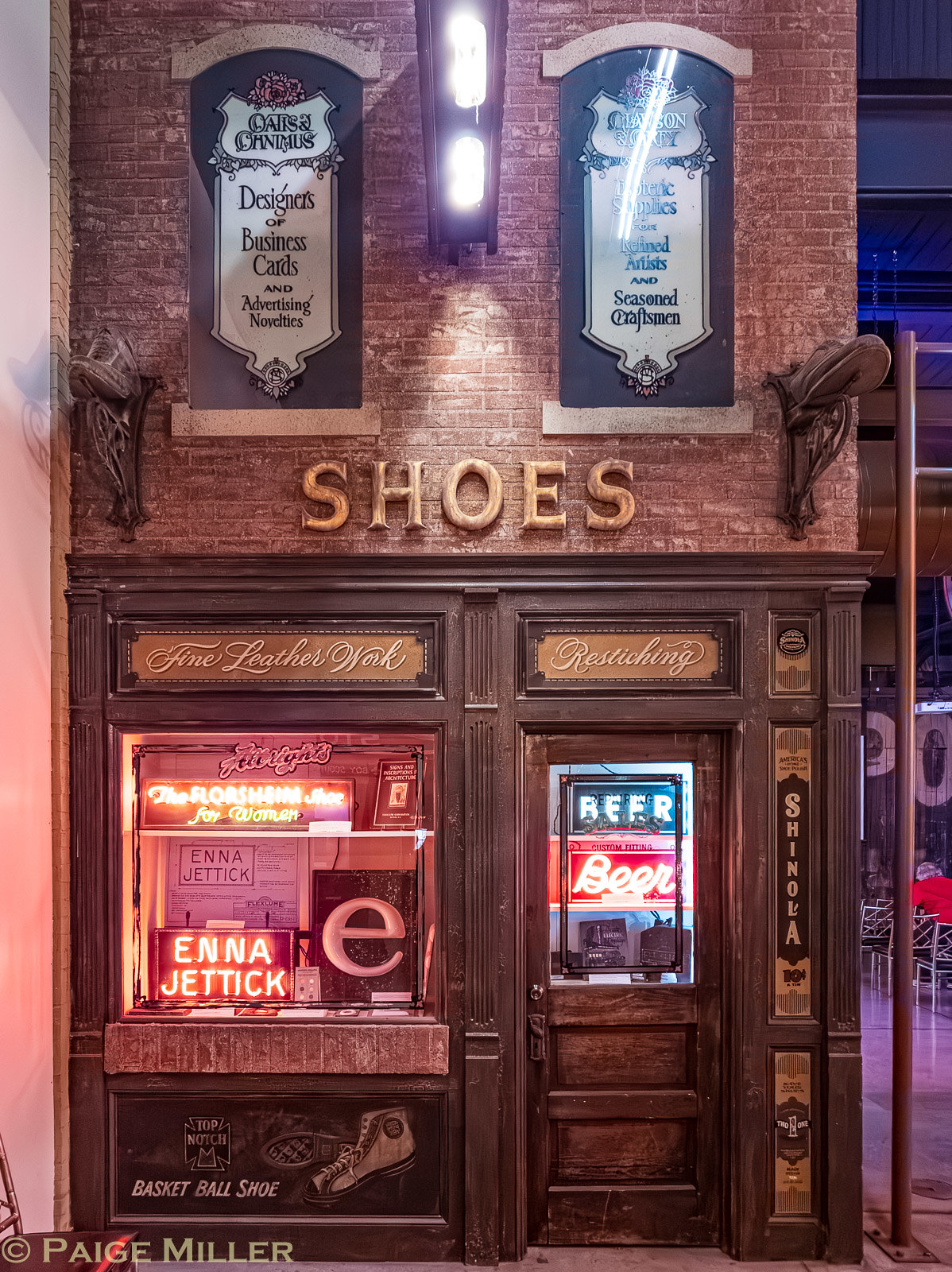The image depicts an intricate, two-story storefront with a blend of old and modern elements. The façade is topped with a red brick wall that boasts two banners in the windows. The left banner reads "Designers of business cards and advertising novelties," while the right reads "Esoteric supplies for refined artists and seasoned craftsmen." The storefront itself is made of carved wood. At the very top, a prominent sign reads "Shoes," flanked by L brackets adorned with shoes.

On the ground level, the forefront features a wooden door with a lit window. Above the door, a sign reads "Restitching." To the left of the door, a main storefront window houses a neon sign that says "Energetic," alongside a square with a pink letter 'E' and another sign for "Energetic" inside the window. The neon lights, although vibrant, obscure some text. The brick wall beneath the windows is illuminated by bright white lights from a brown light casing above.

The storefront includes a vertical sign spelling "Shinola" and neon lights that spell "Beer" in two styles: blue lights on a red background and yellow lights on a blue section. The very bottom left corner bears the copyright "Paige Miller." The scene combines old-style aesthetics with modern touches, giving it a unique, almost reimagined appearance.